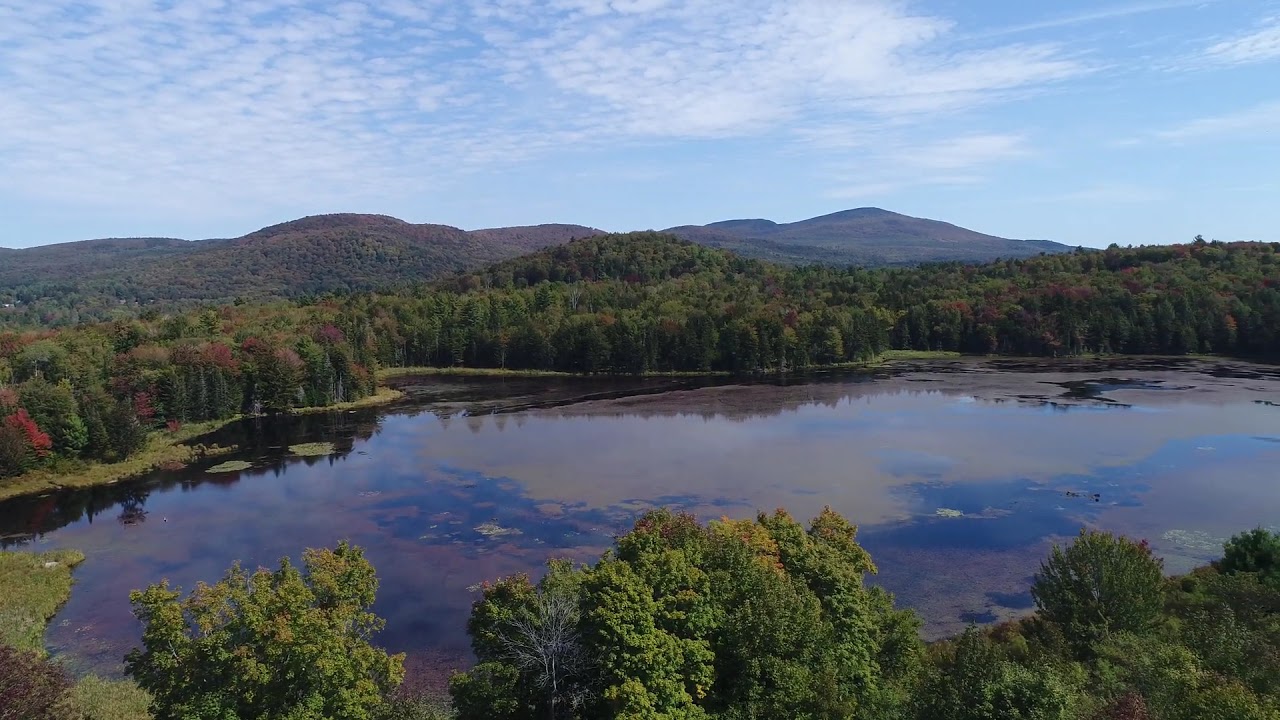This captivating aerial photograph captures a large lake or pond, occupying the image from the bottom left to the right middle. The lake’s surface has patches of algae, adding texture to its otherwise clear reflection of the partly cloudy sky above. In the foreground, a dense line of trees stretches from the left to the right edge of the image, their lush green foliage indicative of late summer with a hint of autumn as some begin to turn shades of orange and red. Beyond the lake, another stretch of verdant trees covers the landscape, giving way to a forested area. This forest extends into rolling hills in the distant background, creating a serene transition from nearby greenery to the low-lying hills, under a canopy of scattered, wispy white clouds in the bright blue sky.